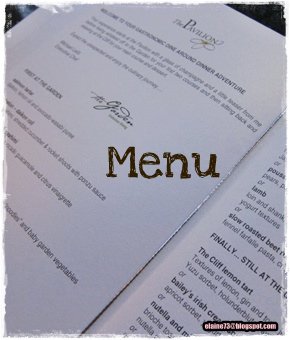This is a detailed photograph of The Pavilion restaurant's menu. The layout features two visible pages with a subtle, shadowed watermark at the bottom in black and white text. At the center of the image, the word "Menu" is prominently displayed in a brown font. Above this, "The Pavilion" is written in a stylish gray font, accompanied by a delicate floral icon situated just beneath the restaurant name.

The menu pages show a variety of dishes, although the text on the left page appears slightly blurry and hard to discern. The right page, however, is clearer and lists several enticing dishes in black font. Notable items include a lamb dish, slow-roast beef, a citrusy cliff lemon tart, a dessert featuring Bailey's Irish Cream, and a Nutella-based product.

The photograph itself has a vintage feel, with an aged effect around the edges that gives the impression of wear and tear, adding to the overall nostalgic and rustic ambiance of the image.